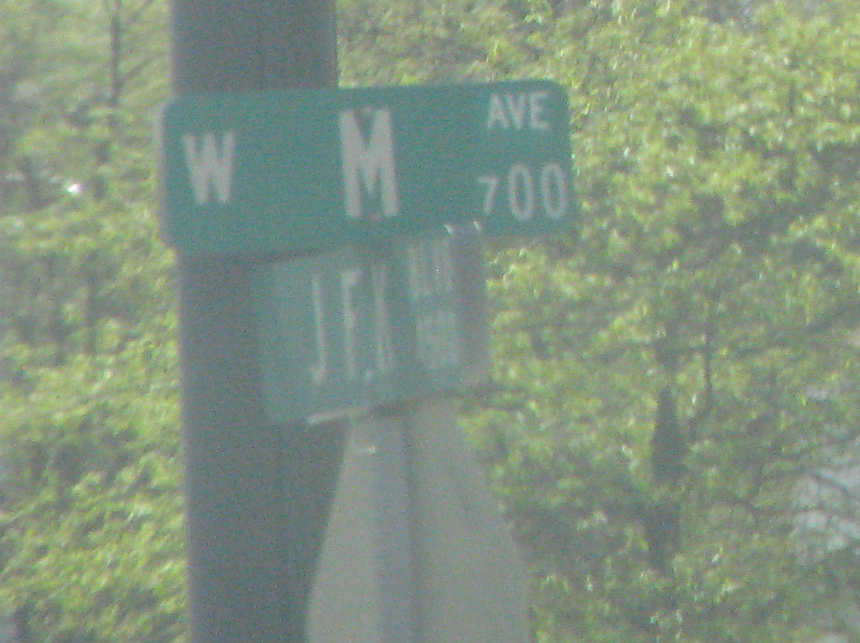The photograph captures a street sign at an intersection, featuring two elongated green signs stacked one above the other. The signs are viewed from an angle, emphasizing their placement at the corner rather than facing directly down either street. The bottom sign reads "JFK Drive," followed by some illegible numbering in white text. Above it, the top sign displays "W M Ave" in white letters, with the numeral "700" where the "7" is noticeably smaller than the subsequent zeros. In the background, there is a thick, dark-colored utility pole, partially obscured by green foliage and the dark bark of tree trunks and branches.